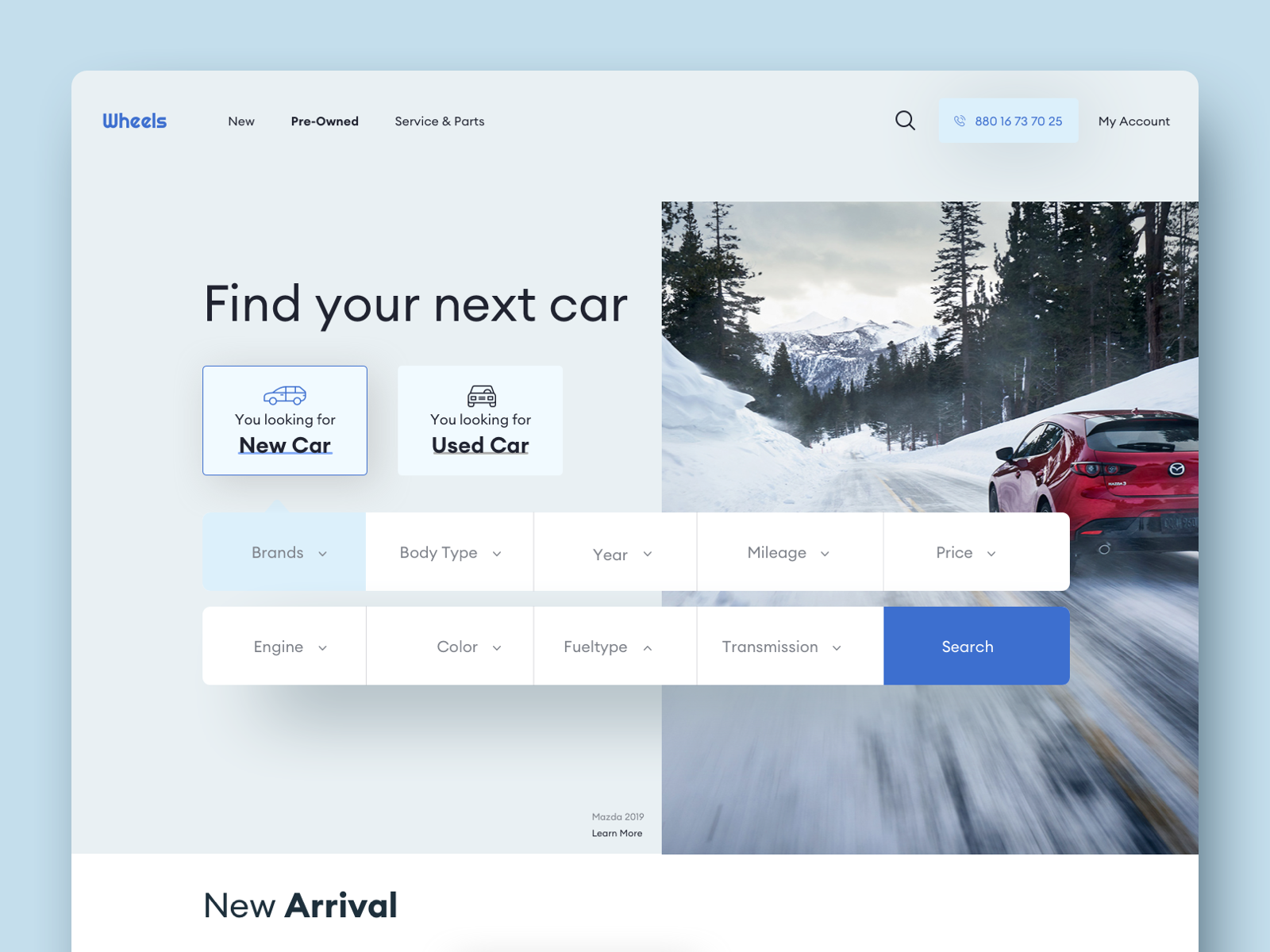The image is a detailed screenshot of a website. The overall website background is light blue, complemented by an embedded image section with a white background. Along the top of this embedded section, the website's navigation bar features blue text on the left that reads "Wheels," followed by black text reading "New," "Pre-Owned," "Services," and "Parts." To the far right, there is a magnifying glass icon representing the search function. Adjacent to this, there's a light blue button with darker blue accents containing the phone number "808-1673-7025," and next to it, black text that says "My Account."

On the right side of the screenshot, the image vividly displays a red car driving up a snowy road. Surrounding the road are snow banks, pine trees, and a distant mountain backdrop, all under a snowy and icy condition. 

On the left side of the image, black text on a white background states, "Find your next car." Below this text are two square buttons; the left one reads "Looking for your new car," and the right one says "Looking for used car." Beneath these buttons is a dropdown menu with various tabs labeled "Brands," "Body Type," "Year," "Mileage," "Price," "Engine," "Color," "Fuel Type," and "Transmission." A blue button labeled "Search" is positioned at the bottom of these tabs. Additionally, beneath this search section, the text "New Arrival" is displayed in black.